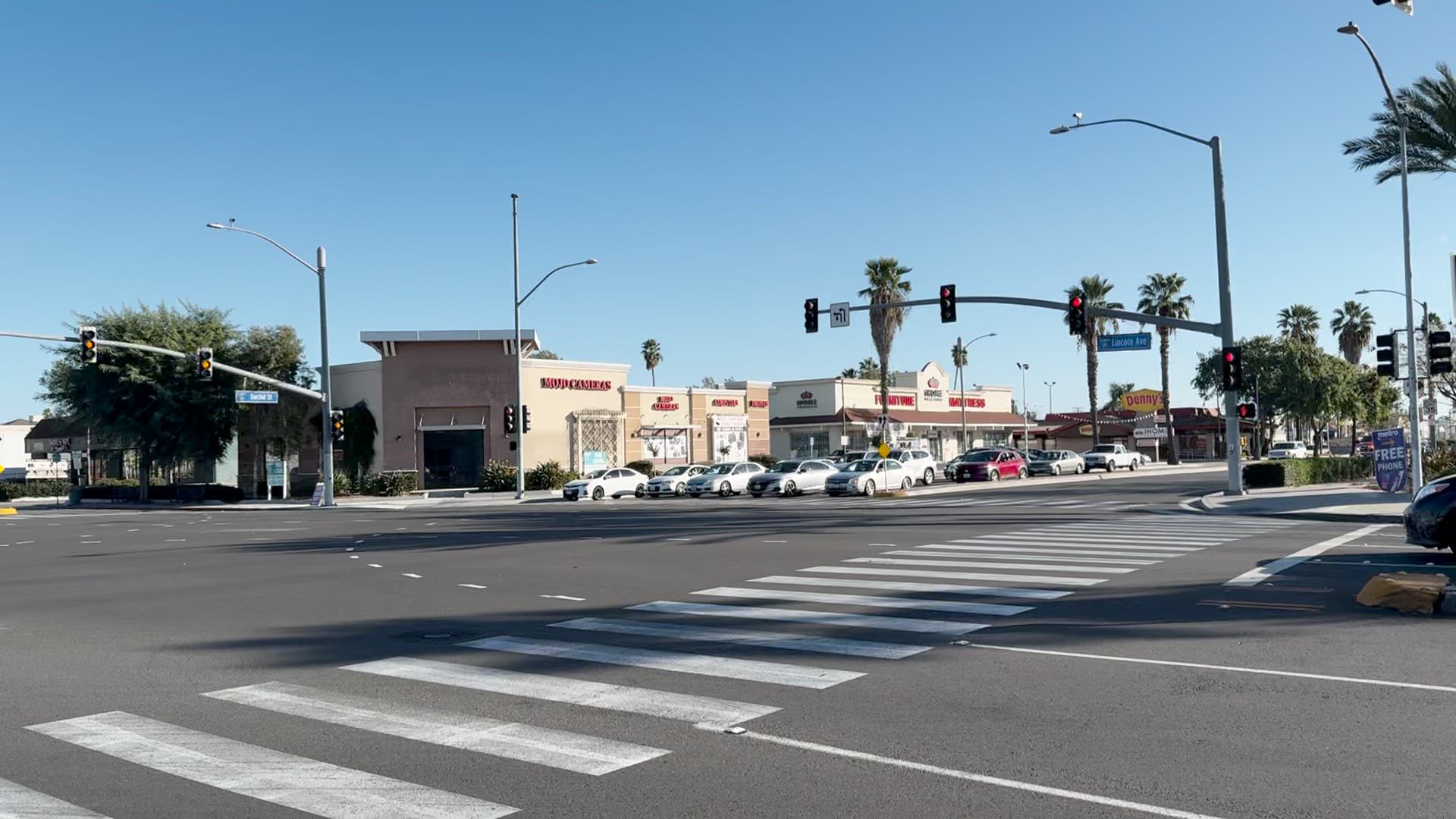The color photograph captures a bustling city street scene. Diagonally across the center of the image stretches a crosswalk laid across the black asphalt. On the left side of the frame, the traffic lights have shifted to yellow. Attached to the traffic light post, a blue street sign is visible, although the inscription is unreadable. Adjacent to the traffic lights stands a tall streetlight, topped with a mounted traffic camera.

In the center of the image, several cars wait at the light, their movement temporarily halted. To their right, various buildings line the street, including one labeled "Mojo Cameras" and another displaying "Furniture Mattress." Some of the signs on the buildings are illegible, but a distinct Denny's restaurant is easily recognizable.

The traffic lights in the middle of the image, governing cross traffic, are currently red. The pedestrian crosswalk sign signals a red hand, indicating that crossing is not permitted. A second tall streetlight bearing another traffic camera is also discernible.

To the right of the image, the front part of a waiting car is visible, paused at the intersection. The sidewalks are lined with numerous trees, predominantly tall palm trees. Above, the sky is a clear, cloudless blue. The dimensions of the photograph are notably wider than it is tall, offering an expansive vista of the urban environment.